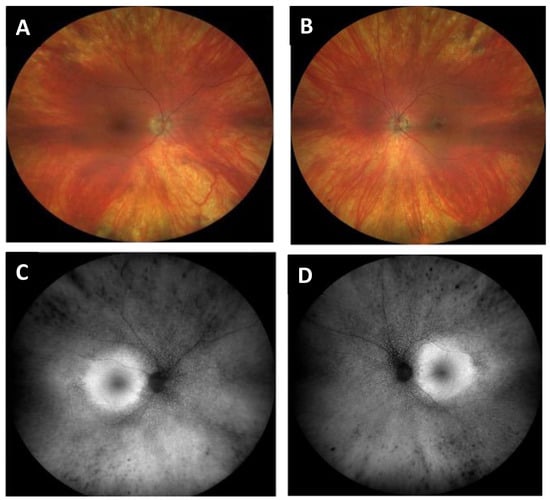The image consists of four microscope views labeled A, B, C, and D. The top two images, A and B, are in color, displaying a vivid scene primarily dominated by red hues that gradually fade into yellow. These images appear circular with a distinct black border. Within these circles, there are white lines and varying shades of red, creating a somewhat "bloody" appearance.

The bottom two images, labeled C and D, are in black and white, providing more detail and contrast. Image C has a prominent white circle situated to the left, with a nearby blood vessel or vein visible on the right side. In image D, the white circle is positioned to the right, with the related blood vessel or vein appearing on the left side. Both black and white images exhibit a central black dot or cell-like structure from which several lines extend towards the circle's edge. This setup makes the black and white images appear illuminated, with a donut-shaped white light surrounding a darker core, intensifying the contrast and detail compared to the color images. Despite the detailed presentation, the exact nature of what is being observed—be it the interior of an eye, a vein, or a general cellular structure—remains unidentified.